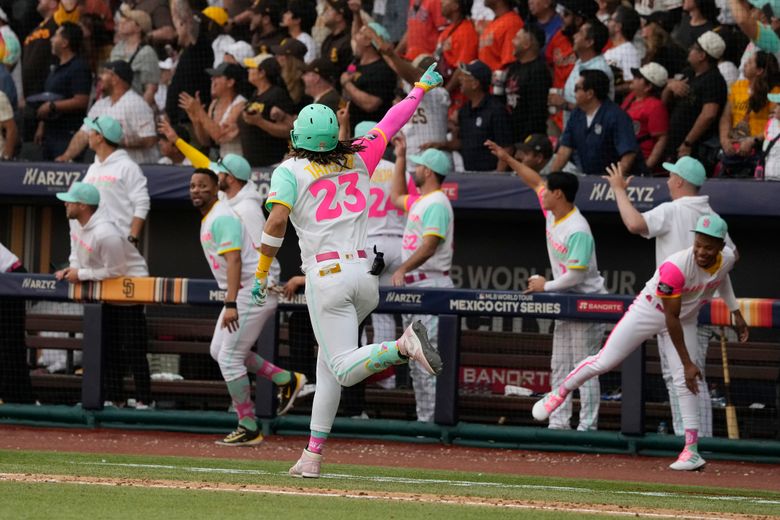The image captures an exhilarating moment during a baseball game at a stadium, part of the Mexico City Series. In the background, a large crowd of enthusiastic spectators is seen, all focusing towards their right, clapping, shouting, and cheering energetically. Their excitement is palpable as they witness a significant event unfolding on the field. In the middle ground, the players' dugout is bustling with activity. The team, dressed in white uniforms accented with pink neon and yellow details, along with green batting helmets, are predominantly dark-skinned and appear jubilant. A player, who seems to have scored, is in the foreground, running with one leg up and the other on the ground, pointing towards the audience, celebrating the victory. His green helmet contrasts with his red hair beneath it. Coaches and reserve players are also present in the dugout, contributing to the celebratory atmosphere. The sun shines brightly, indicating a warm day, as everyone revels in the moment of triumph.